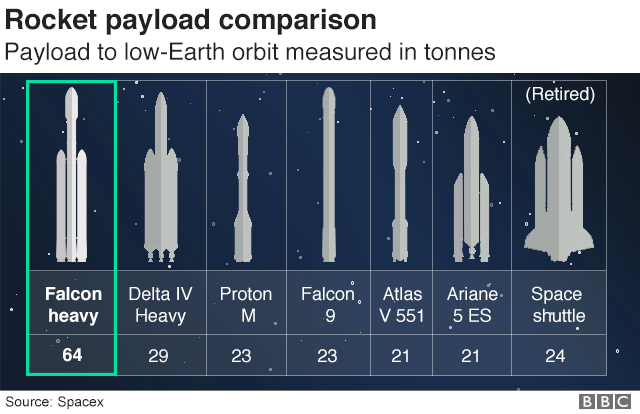The image depicts a detailed chart titled "Rocket Payload Comparison" set against a dark blue or black background with white dots simulating stars. It compares the payload capacities to low Earth orbit, measured in tons, of seven rockets. The chart features simple rocket silhouettes, half dark gray and half light gray, arranged from left to right. The rockets are labeled as follows: Falcon Heavy with a payload of 64 tons (outlined in green), Delta IV Heavy with 29 tons, Proton M with 23 tons, Falcon 9 with 23 tons, Atlas V 551 with 21 tons, Ariane 5 ES with 21 tons, and the Space Shuttle with 24 tons, the latter marked as retired. Additional text includes "Payload to Low Earth Orbit Measured in Tonnes" and sources listed as SpaceX on the lower left and BBC on the lower right.